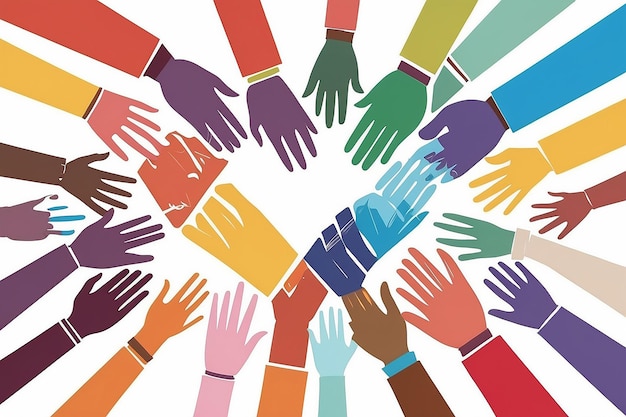The vibrant rectangular digital artwork, approximately four inches wide and three inches high, features a plain white background from which numerous multicolored hands and forearms extend from every corner toward the center. These hands, depicted in a riot of colors including brown, blue, orange, pink, magenta, green, yellow-toned mauve, and more, create an intricate network of reaching limbs. Each forearm is clad in a long-sleeved shirt with a variety of colored cuffs, contrasting beautifully against the hands. Despite the vibrancy, the image exhibits some distortions—such as abnormally long fingers and a purple hand with only three partially blue fingers—suggesting it might be AI-generated. Notably, in the top left, an oddly proportioned hand has a ring finger and index finger of equal length. At the center, two distorted hands form a V shape, with the left hand appearing to hold an indistinct object. These central hands and the overall jumbled appearance evoke a sense of chaotic energy, exacerbated by the bright colors and varied forms.